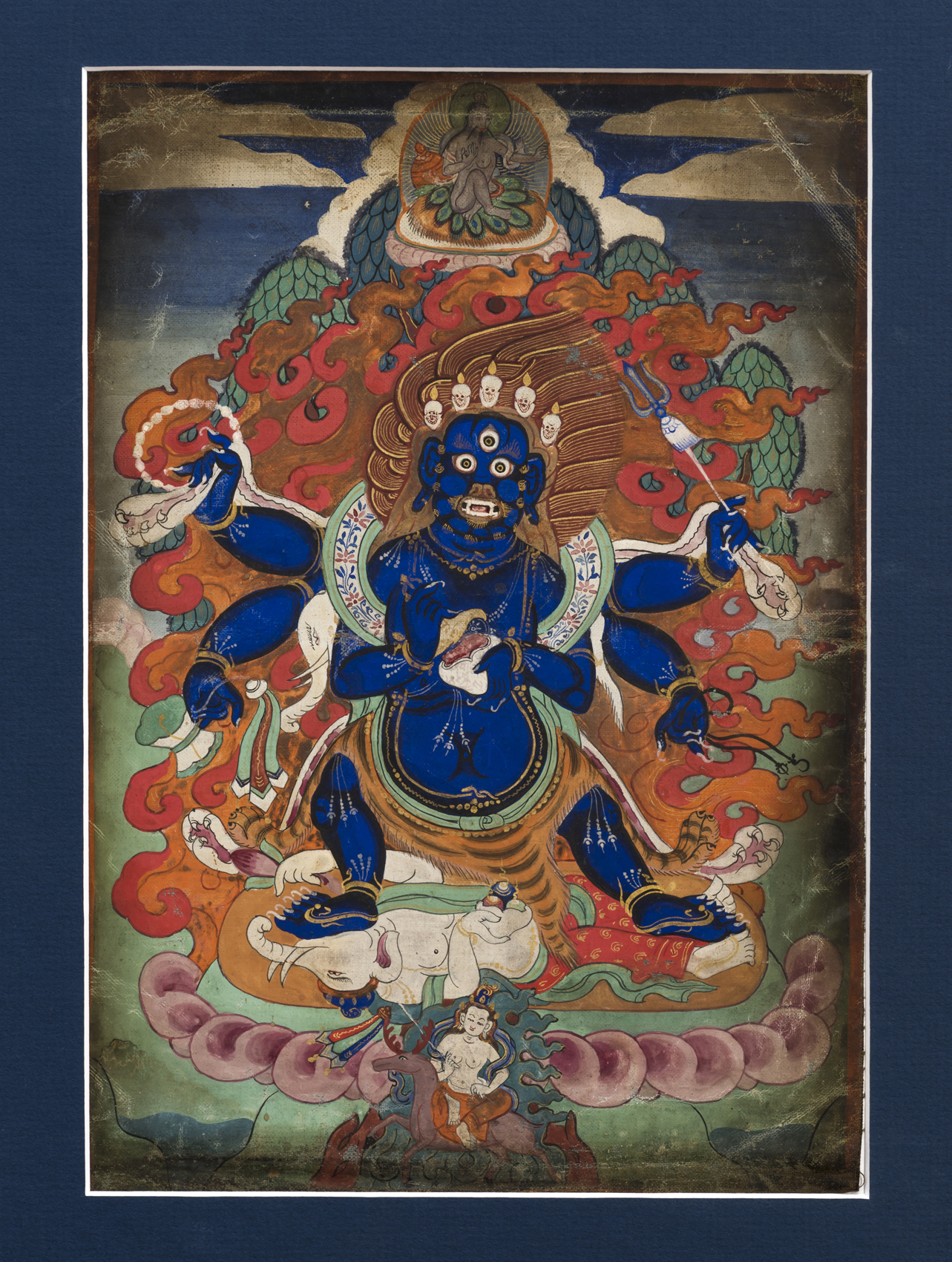The detailed image depicts a colorful and intricate portrayal of a blue deity, likely of Tibetan or Hindu origin. The central figure, humanoid in form, exhibits three eyes - one positioned on its forehead along with two in traditional placements. It has six arms and two legs, adorned with short, white fingernails or claws. Each arm holds distinct objects: one arm clutches a trident with a white tassel, another a string or cord with a sickle and smaller trident, while others hold items resembling a meat fork, a wand-like object, and what might be a monster paw necklace and a mallet. The deity's attire includes a distinct tiger-striped loincloth and a rounded collar with blue, white, and red floral designs bordered in light green.

The deity stands atop an upside-down elephant-headed figure wearing red baggy pants and a green sash. Below this figure, there is another smaller character with green flame-like elements around them, clad only in an orange robe. Another person depicted towards the back is nude, has a halo, and stands on a gold mound adorned with green leaves. The scene is surrounded by fiery, golden-red designs, and at the top, a dark blue sky embellished with stylized white clouds and pink, smoke-like forms can be seen. A figure sits atop this sky scene on what appears to be a bed of peacock feathers. The entire composition has a blue border, with the lower section featuring pink and blue shapes surrounded by green bow-like figures, resembling leaves or scaled motifs.